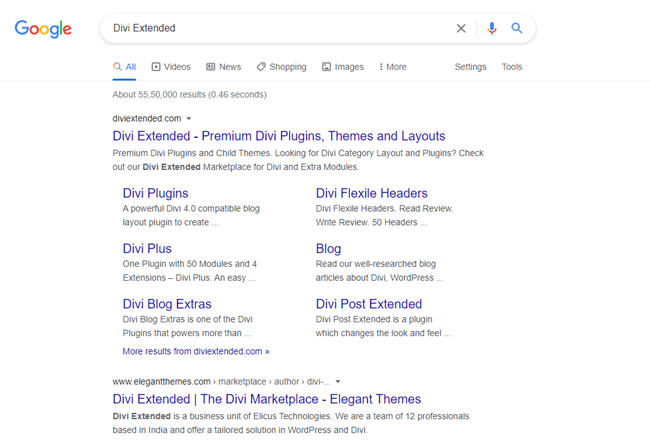A detailed caption for the image:

"Explore the comprehensive offerings of Divi Extended, the premier marketplace for Divi and Extra modules, plugins, themes, and layouts. Powered by elegant themes, Divi Extended provides premium Divi plugins like Divi Flexible Headers and Divi Plus, which effortlessly extend the capabilities of your Divi website. Visit diviextended.com for a wide array of Divi category plugins and trial themes, perfect for enhancing your WordPress site. Check out our well-researched blog articles for in-depth insights on Divi WordPress and the latest plugin updates. Serving a dual-person base in India, Divi Extended offers tailored solutions for all your WordPress needs."